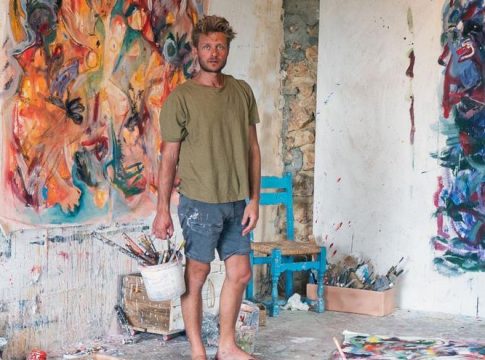The image depicts a man standing in an art studio, surrounded by vibrant, abstract murals. He is dressed in a brown (or hunter green) T-shirt and blue shorts that are flecked with paint. In his hand, he holds a white bucket filled with paintbrushes, some of which have colorful tips. To his right, there's a blue wooden stool next to a box brimming with additional brushes, and a second box is visible to the left of the stool. The studio floor is cluttered with various painting supplies. The left wall behind him features a mural dominated by warm colors such as orange and yellow, while the right wall displays a mural with cooler hues like blue, purple, and red. The background includes white-painted walls, with one corner adorned by a small table or object that's difficult to discern. The floor seems to be cement gray, and there are hints of other artistic elements and textures throughout the space, including a possible depiction of a fence or rocky wall.